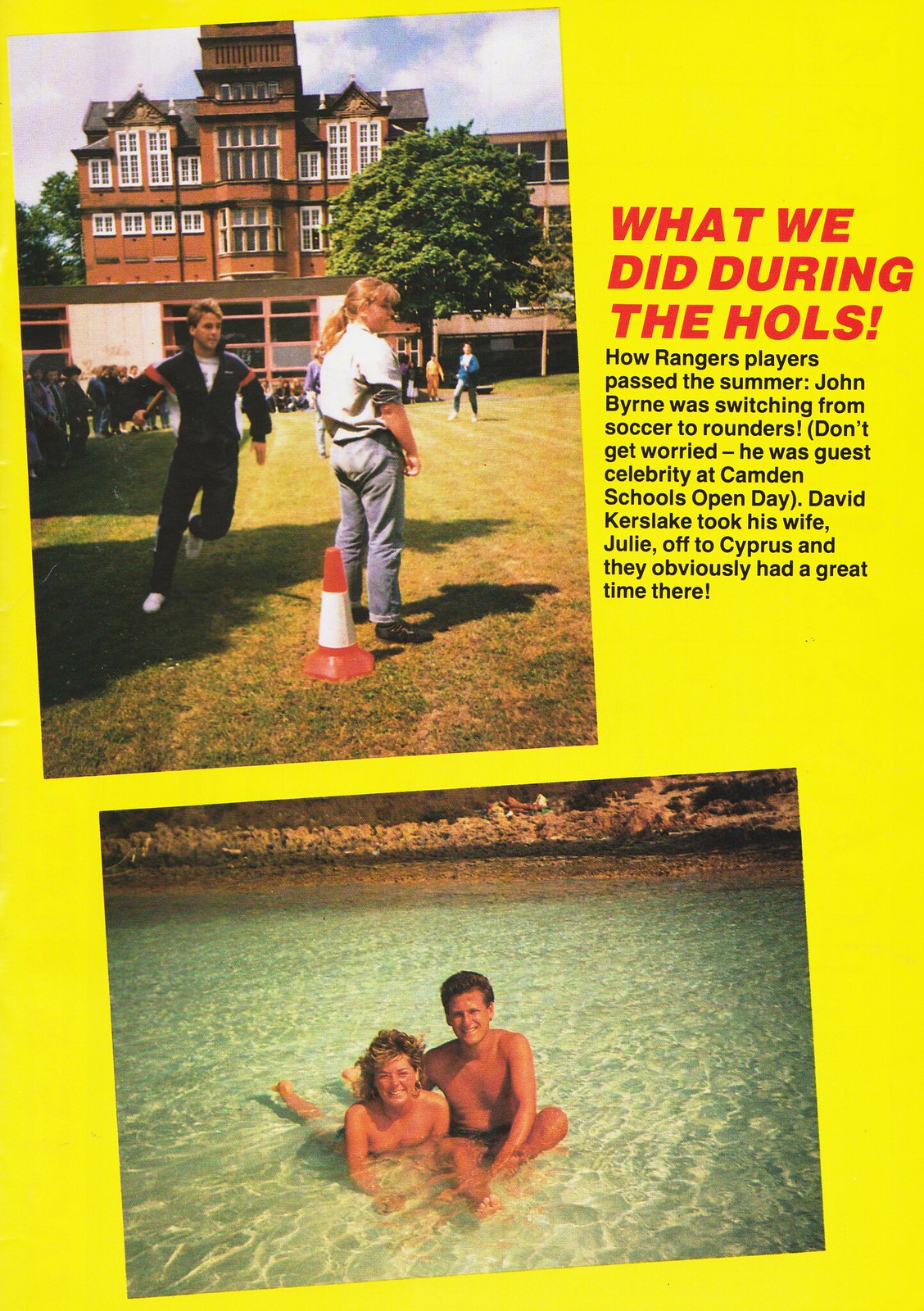The image features a vibrant yellow background with two photographs, each slightly angled to the left, creating a dynamic composition reminiscent of a sports magazine's entertainment section. At the top left, a portrait-oriented photo showcases a grassy field bustling with activity. A man in a black tracksuit is captured mid-run, while a woman in blue jeans stands nearby, looking to the right. An orange cone is visible behind her, and in the background, a multi-story brick building looms under a sky dotted with clouds. Scattered across the field are various people engaged in different activities.

Below, a landscape-oriented photo depicts a man and a woman in bathing suits, smiling as they recline in the shallow water, their arms around each other. The woman has brown hair and a tan complexion, while the man, also tan, sports dark hair.

In the upper right corner of the image, red text boldly states, "What We Did During the Halls!" Below, in black print, a paragraph elaborates on the summer activities of Rangers players. It reveals that John Byrne transitioned from soccer to rounders as a guest celebrity at Camden School's Open Day, while David Kerslake enjoyed a joyful trip to Cyprus with his wife Julie, who is featured in the bottom photograph. The overall style combines photographic realism with graphic design elements, resulting in an informative and visually engaging presentation.